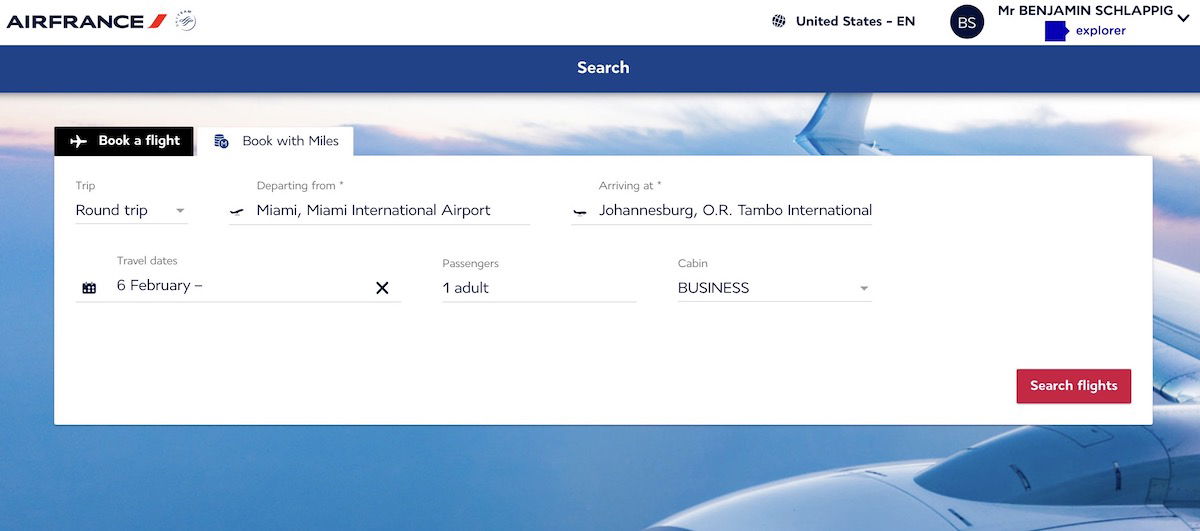The image displays a detailed interface of an online booking system for Air France. 

At the top, the Air France logo is featured prominently with a red diagonal line next to it. To its right, there is a light gray circle adorned with small notches around its edges, though the exact content in the middle of the circle is indistinguishable. Further to the right, there is a text reading "United States-EN" alongside a small blue circle containing unclear letters or numbers. Below this, the name "Mr. Benjamin SCHLAPPIG" is displayed.

To the right of the name, a blue square with a small triangle on the right end is labeled "Explorer." Beneath this is a prominent blue bar labeled "Search and Wait." Below the bar, an image of an airplane flying against a sky backdrop is showcased. Further down, a black rectangle with white text reads "Book a Flight," next to a white rectangle with black text and blue elements which reads "Book with Miles."

The main section contains a large white rectangular area categorized under "Trip." It includes details for a "Round Trip" originating from "Miami, Miami International Airport" and arriving at "Johannesburg O.R. Tambo International." There are additional words that are not fully legible, with a sequence of three distinct elements beneath them. Another box with dotted borders is labeled "6 February," followed by a dash, an "X," and the text "One Adult and Business," with gray lines under each term.

In the lower right-hand corner, a red rectangle boldly states "Search Flights."